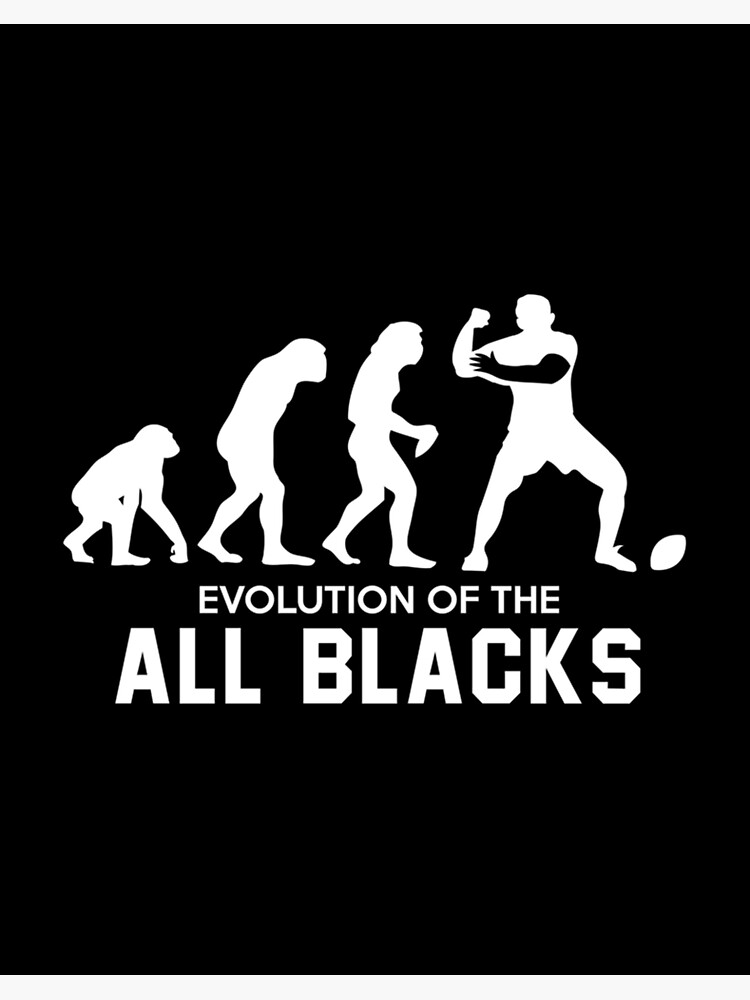The image features a black background with contrasting white silhouettes and text. It portrays the evolution from an ape to a modern human over four stages. The first silhouette depicts a chimpanzee, transitioning into a more upright monkey in the second. The third shows a caveman-like figure, and the final silhouette illustrates a human male, notable for having one black arm, wearing shoes, and preparing to kick a football positioned near his foot. This sequence is captioned "Evolution of the All Blacks" in white text beneath the figures, potentially referencing a sports team. The entire composition is starkly black and white, resembling a poster.